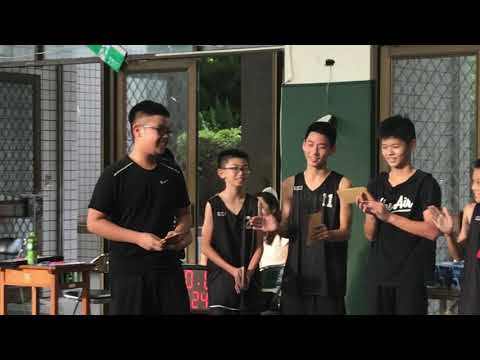The image depicts a lively, indoor gathering featuring five young Asian men and a boy, all clad in black attire, with at least two sporting basketball jerseys, suggesting athletic involvement. They stand side by side, surrounded by the warm ambiance of natural light filtering into the room. The tallest boy, wearing glasses and holding something in his hands, appears to be the center of attention, with the others clapping and smiling towards him, possibly celebrating his achievement or participation in a recent competition or event. The backdrop includes a wall fitted with chicken wire panels and a green-painted section, while an end table resides on the left. The group's joyful expressions and gestures convey a sense of camaraderie, making it a moment of shared celebration in a versatile setting, possibly a venue that opens to the outdoors.